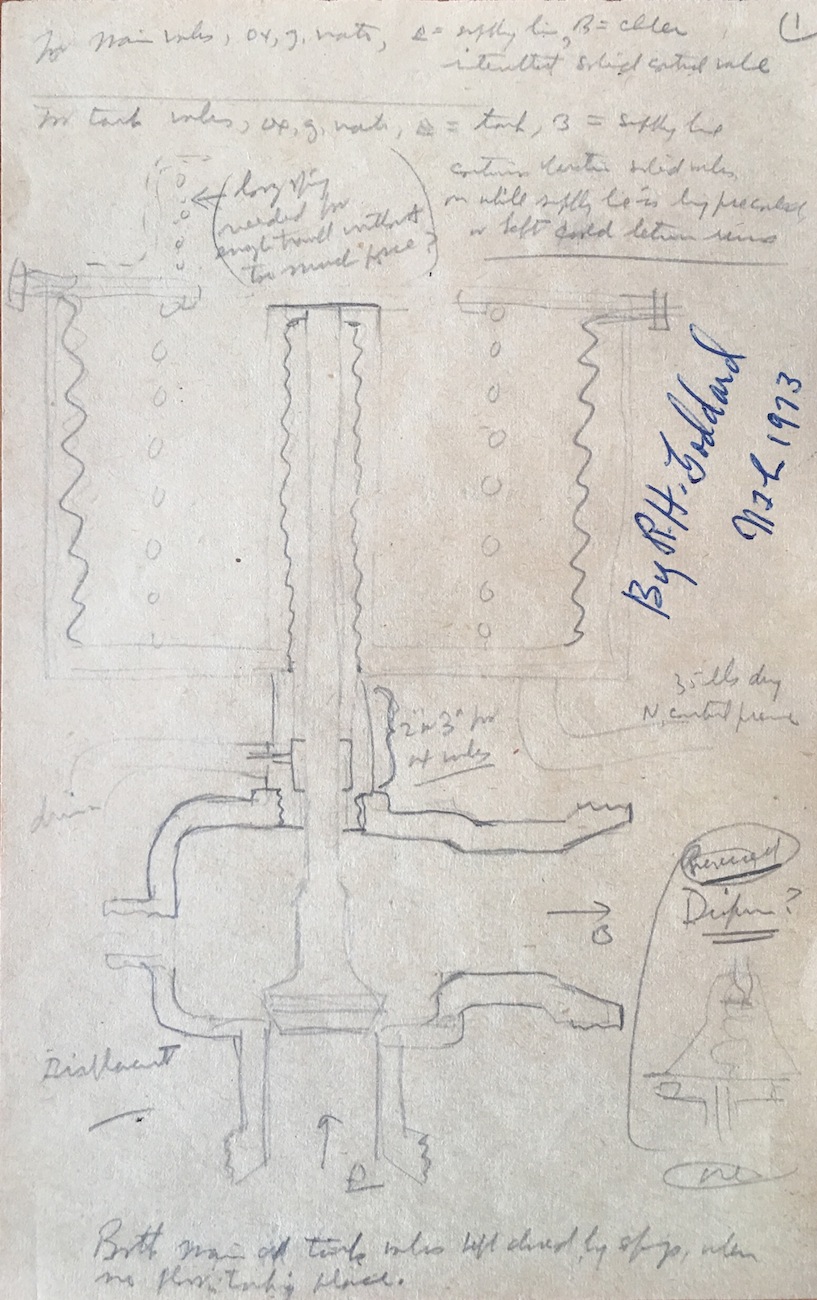This image depicts a detailed hand-drawn engineering diagram on light gray-blue paper. The pencil sketch intricately illustrates a compression-type device integrated within a metal piping system, likely designed for an underground installation. The piping configuration includes sections that curve downwards, extends to the left, then down again, and finally to the right, mirroring the same pattern in reverse at the bottom. The drawing includes various technical specifications and schematics, supplemented by graphs and hard-to-read handwritten notes in cursive. A prominent section on the middle right side features annotations in blue ink, including the name "R.H. Goddard" and the date "1973," though the clarity of some characters and numbers is compromised by the cursive handwriting. This diagram showcases the functionality and intended use of the device it represents, as conceptualized by Goddard in 1973.